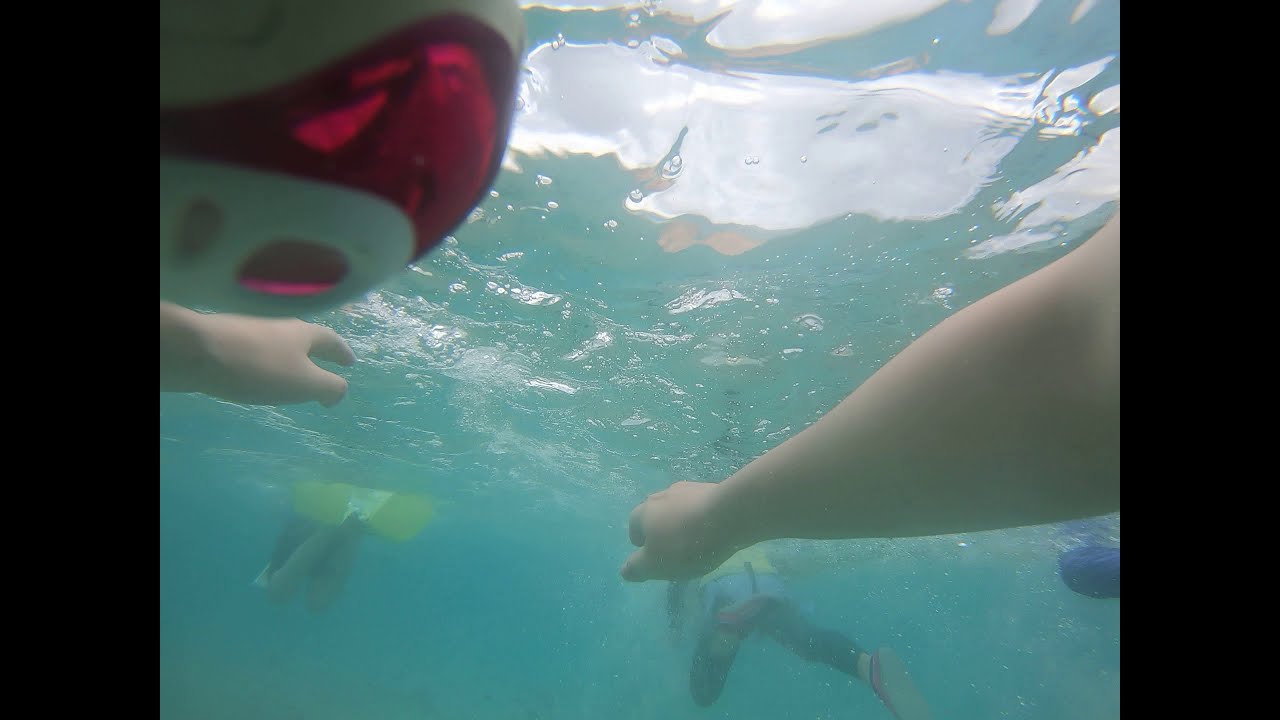This vibrant underwater photograph captures a dynamic scene full of action and color. The image, likely a still from a video, is taken from the perspective of a swimmer, whose outstretched arms frame the right and left sides of the photo. The water is a striking turquoise blue, filled with bubbles and disturbances, indicating movement. Towards the top part of the image, the surface of the water looks glossy and shiny, with patches of white caused by sunlight penetrating the water. Distorted images hint at a bright, sunny day above.

In the upper left corner, a pink-magneta and white flotation device or ball adds a burst of color to the scene. Two people are visible in the frame, swimming ahead of the photographer. One swimmer is noticeable for their pink sneakers, adding a unique touch, while another on the right dons a green and blue top with black pants. Additional colors, including aqua blue, dark pink, lime yellow, light blue, dark blue, and tan, contribute to the rich palette of the image.

The photograph is bounded by thicker black bars on the right and left, suggesting it might be a still from a video. The overall playful yet immersive snapshot captures the essence of being underwater, with sunlight filtering through the water, creating a shimmering effect, and encapsulating a moment of lively aquatic activity.